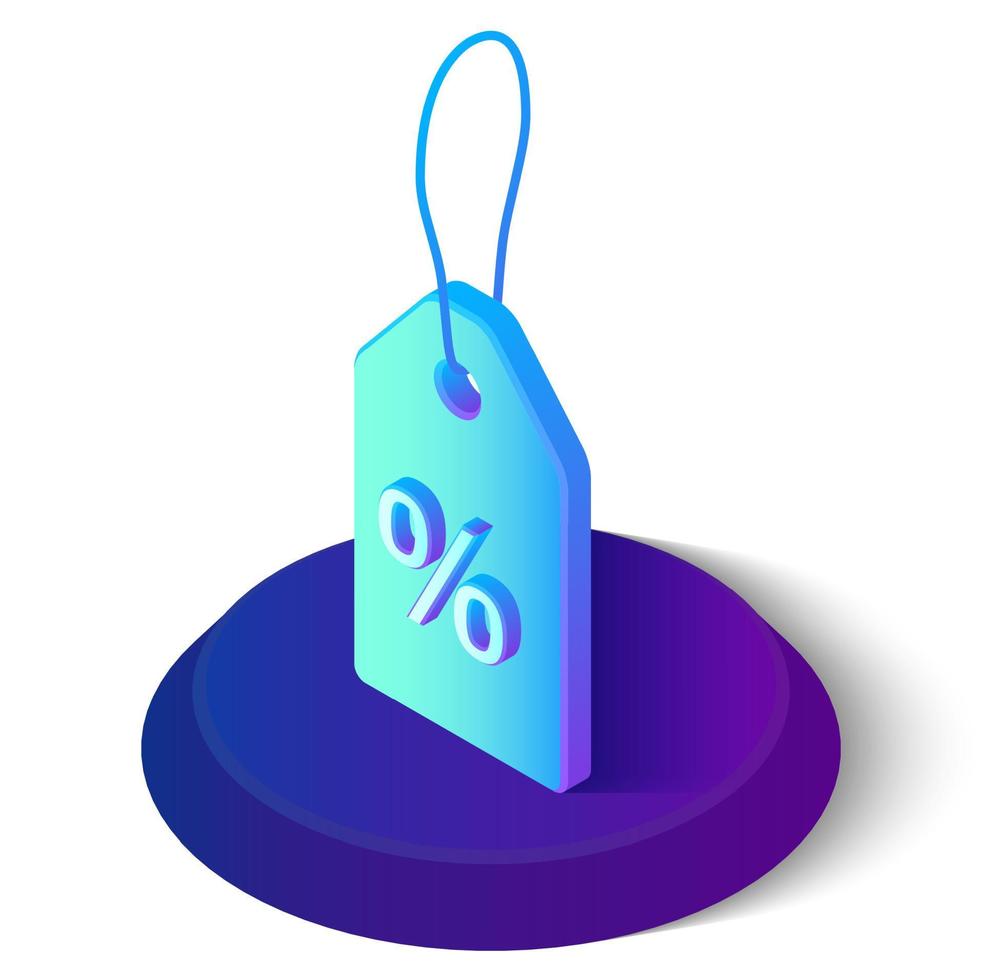On a white background, the image features a three-dimensional blue-violet pedestal with a sloped downward edge and a smaller top compared to its base. Atop this pedestal sits a light blue price tag, designed with a dark blue string and a central dark blue hole at the top. The tag is oriented diagonally and has a percentage symbol (%) in aqua color, with dark blue shadows giving it a 3D effect. The pedestal exhibits a gradient color pattern ranging from deep blue and purple on one end to a lighter, Barney-colored purple on the other. The left side of the tag is illuminated, casting a dark shadow to the right of both the tag and the pedestal. The overall composition is detailed with continuous blue and violet hues that merge seamlessly along their borders.